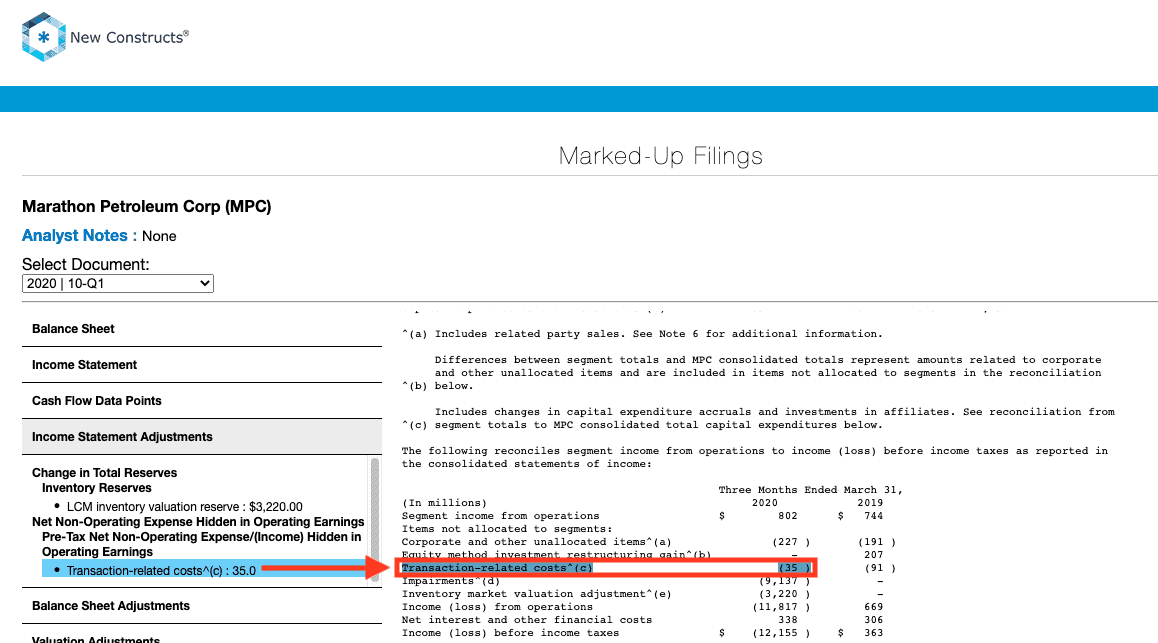**Detailed Caption:**

The image comprises several elements organized systematically within a document. 

- **Top Left Corner:** The phrase "New Construct" is prominently displayed.
- **Central Graphic:** An octagonal shape in blue houses a blue star. Beneath this, a horizontal blue line runs across the image.
- **Main Heading:** Below the blue line, at the center, it reads "Marked-Up Feelings" in black text.
- **Left Section of the Image:** It features a heading, "Marathon Petroleum Corp NPC Analysis Note." Here, "Analysis Note" is highlighted in blue, while the rest of the text remains black.
- **Document Details:** The document is titled "2020 10-Q1," covering various financial statements, including the balance sheet, income sheet, cash flow data point, and income statement adjustments.
- **Highlighted Annotation:** A highlighted note emphasizes a change in total reserves: "Inventory Reserve LLCM Inventory Valuation Reserve $3,220." It further elaborates on "Nest Nine Operating Expense Hidden in Operating Earnings Pretext" and lists "Nest Nine Operating Expense or Income Hidden Operating Earnings Transactions Related Costs." The figure "35" is involved.
- **Arrow & Highlighted Text:** A red arrow originates from this highlighted text, pointing rightward towards another text outlined in red— "Transactions Related Cost 35."
- **Right Section of the Image:** A subtitle, "Balance Sheet Adjustment Valuation Adjustment," sets the theme for the detailed data in the central part of the image.
- **Central Text Block:** The central text block mentions a PC-A included related party, sales data, and differentiation between segment income versus NPC consolidated totals. It outlines significant points like unallocated items and capital expenditures reconciling segment reports with NPC consolidated totals.
- **Table/Spreadsheet:** The lower portion of the image contains a table titled "Three Months Ended." This table, measured in millions, breaks down segment income from operations, unallocated items, equity method investments, restructuring gains, transition-related costs, impairment, venture markets valuation adjustments, net interest, financial costs, and income losses before income taxes.

Overall, the image serves as a detailed financial analytical note for Marathon Petroleum Corp, highlighting specific adjustments, costs, and reconciliations within their financial statements.